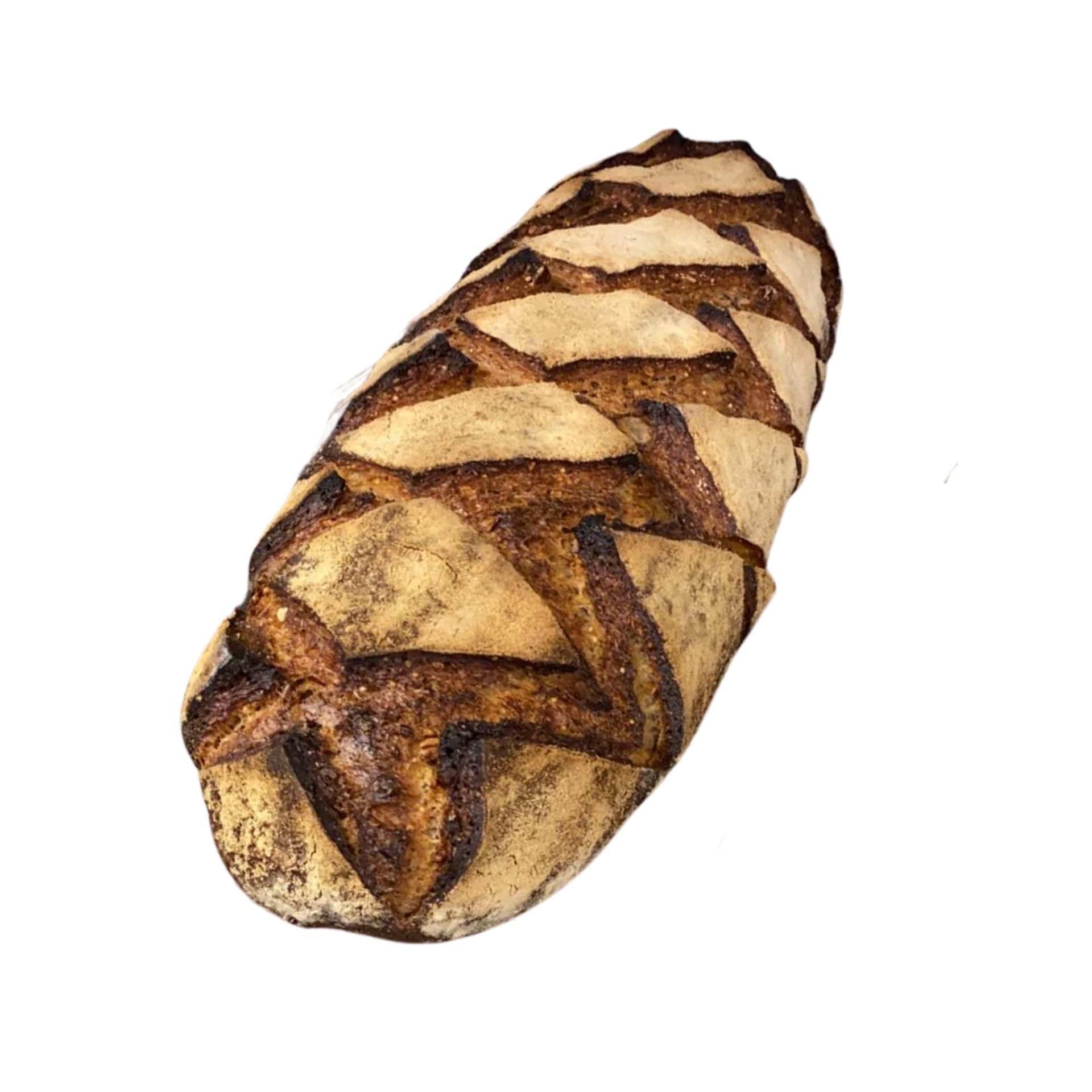This photograph depicts a meticulously crafted loaf of bread, shaped like a long, oblong, and slightly tapered baguette. The loaf has a visually striking crisscross pattern created by deep, dark brown, crusty score marks against a lighter tan background, speckled with some dark spots. This artisanal bread showcases a diamond pattern across its surface, indicating a careful and creative hand in its preparation. The loaf is presented at an angle, ascending diagonally to the right, emphasizing its substantial size and appealing texture. This image exudes a rustic, homemade charm and would be perfectly suited for showcasing on a website or as part of a stock photo collection.